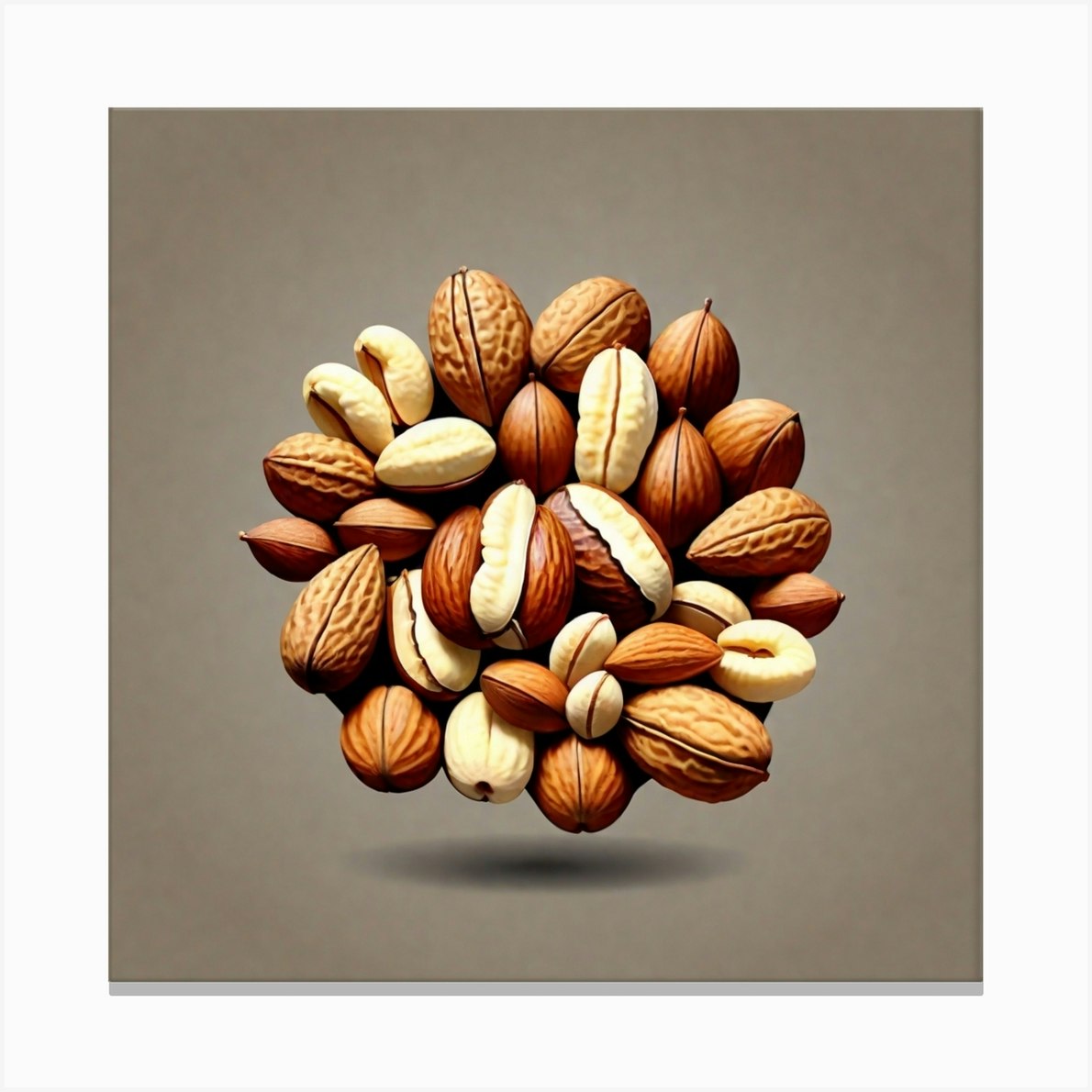The image features an artistic rendition of various nuts, intricately arranged to form a circular, flower-like pattern at the center. The nuts, including macadamia nuts, almonds, walnuts, cashews, hazelnuts, and Brazil nuts, appear to be floating, casting a light, oval shadow beneath them. This gives the impression of them hovering against a slate grayish to beige, khaki-toned background. The arrangement and coloring, ranging from light yellow to tan to chestnut brown, create an impression of a unified bouquet of mixed nuts and shells. The detailed depiction suggests a blend of photographic realism and painting, presenting a visually appealing cluster that celebrates the growth and diversity of nuts.